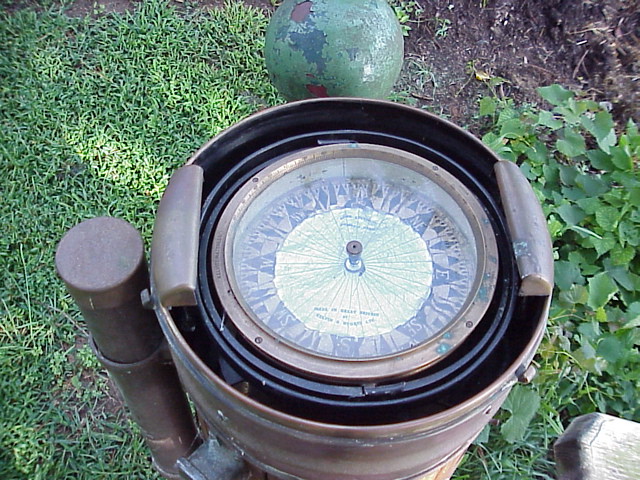This color photograph depicts a detailed close-up of a vintage compass housed in a copper, light brown, and dark brown metallic container. The round compass is recessed into this metallic housing, leaving a visible space around its edges. The outer rim of the compass features two black concentric circles. The main face of the compass is copper-toned and highly ornate, displaying cardinal and intercardinal directions — north, east, southeast, south — along its light brown and black-trimmed border.

The ornate border includes intricate black triangles and rectangles. Radiating from the center to the border, light green lines contrast against the beige background, leading to a central metallic knob. The compass is mounted on a cylindrical metallic post elevating it off the ground. Surrounding the base is short grass and a small bush with green leaves positioned on the right-hand side. In the background, a distressed green sphere with chipped dark green and light blue paint appears near the compass, although it is unclear whether it is attached to the compass or simply lying on the ground.